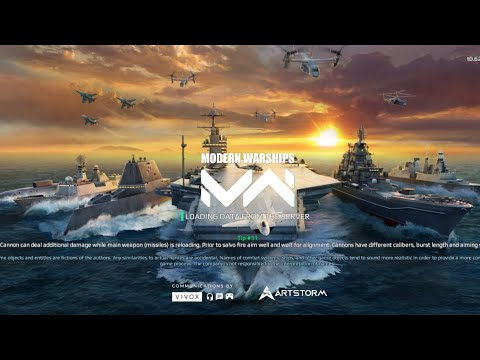The image depicts a loading screen from the video game "Modern Warships" developed by ArtStorm, featuring a logo that combines the letters "M" and "W" prominently in white font at the center. Below the logo, the text states "Loading data from the server." The background showcases an ocean scene at either sunset or sunrise, characterized by a cloudy sky with hues of gray and yellow, and bright sunlight to the left. Five military battleships dominate the foreground, with ocean waves lapping against their sides, and they appear to be advancing towards the viewer. The sky above is crowded with an array of military aircraft, including fighter jets, large helicopters, and Ospreys. The image also includes a tip at the bottom in green font, with text that's partially obscured due to quality, likely suggesting strategic advice for gameplay; it reads "Tip number 11." Additional textual elements note support features like VIVOX and a depiction of a headset and game controller, alongside an arrow pointing upward with the label "ArtStorm." The picture is bordered by black bars at the top and bottom.